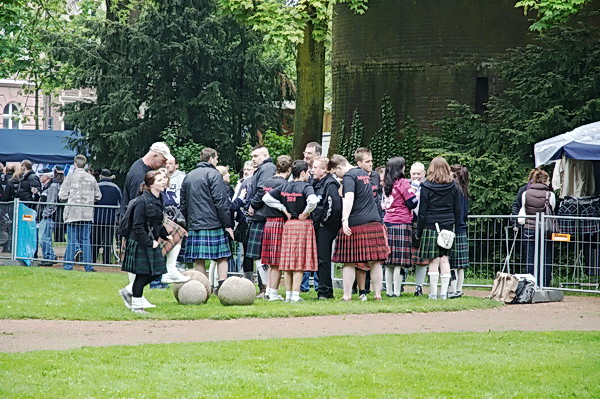The image portrays a large group of people gathered in a grassy field, forming an almost circular huddle. Most of them are wearing black shirts with red writing and plaid kilts in colors such as red, blue, and green, that fall below their knees. In front of the group, there are two stone-like concrete spheres, adding a distinct texture to the setting. The background features a metal fence separating this group from additional tents and other individuals who are not wearing kilts but are dressed in long sleeves and long pants. Adding to the picturesque scene, there is a structure resembling a castle tower with vines climbing up its stone walls on the right side, and a large tree standing majestically to the left. The overall ambiance and elements suggest that this could be a festival or a cultural gathering set in a park with patches of green grass interspersed with concrete paths.